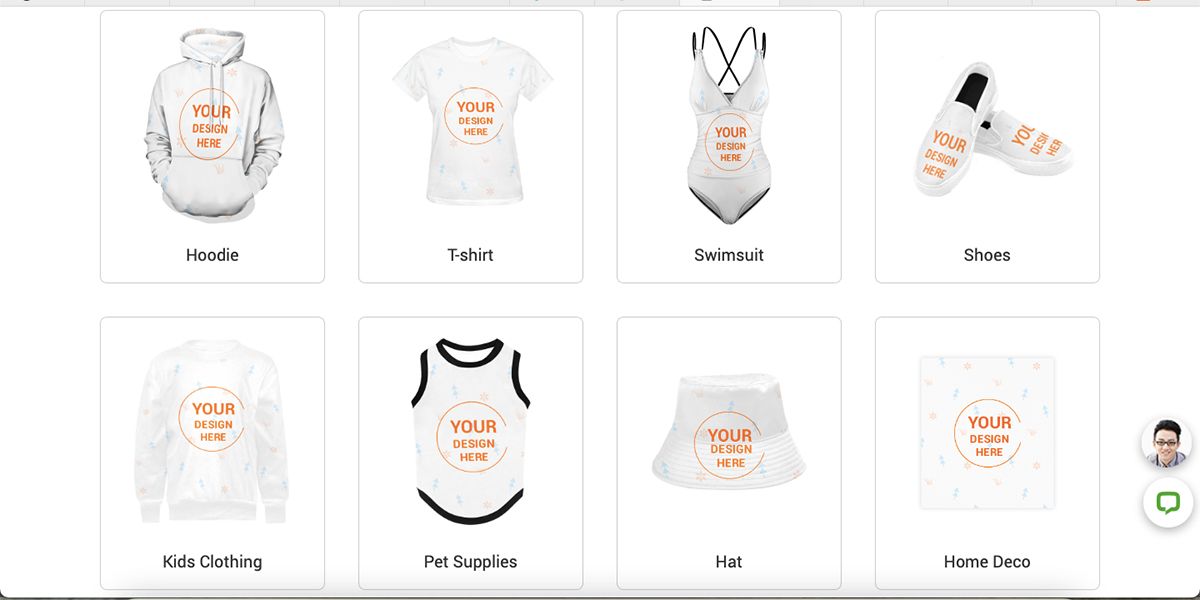A detailed and descriptive caption for the image:

The image depicts a grid layout of eight custom-made clothing and accessory items, each displayed in individual boxes against a white background. Each item prominently features a central logo in the form of an orange circle with the text "Your Design Here" in capital letters.

Starting from the top row, left to right:
1. A white hoodie labeled "Hoodie."
2. A white t-shirt labeled "T-shirt."
3. A white swimsuit labeled "Swimsuit."
4. A pair of white canvas loafers labeled "Shoes."

On the bottom row, left to right:
1. A white children's sweatshirt labeled "Kids Clothing."
2. A white pet shirt with black trim, likely for a dog, labeled "Pet Supplies."
3. A white hat resembling a casual beach hat, labeled "Hat."
4. A white tablecloth labeled "Home Deco."

To the right of the grid, there is an illustration of a profile picture depicting a character with dark hair and glasses. Below this illustration is a chat bot button, offering an interactive chat option on the site.